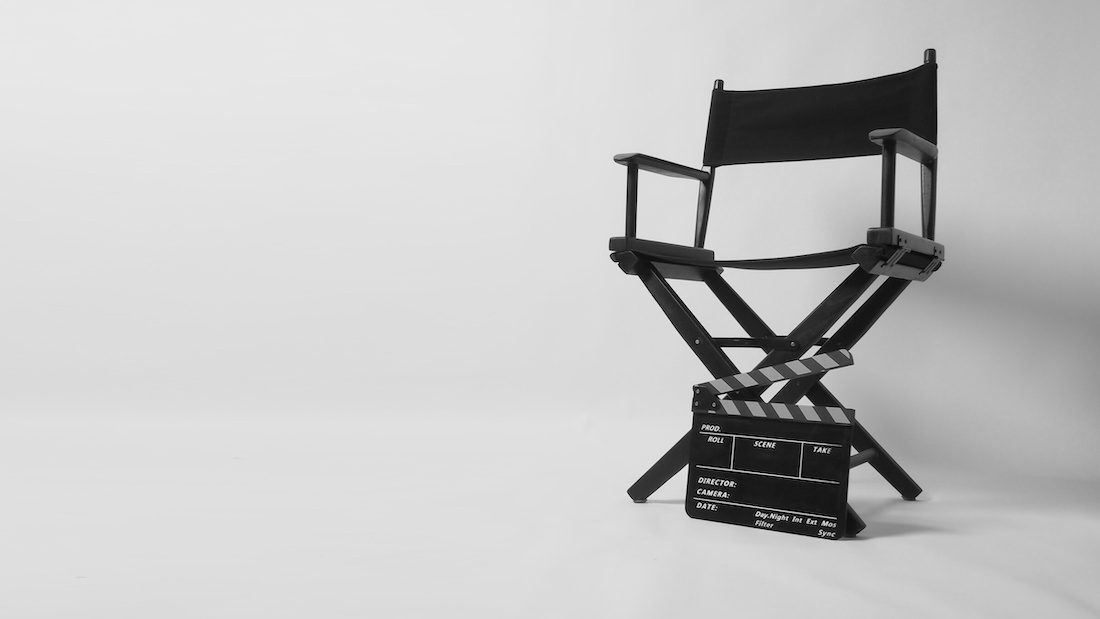The photograph features a classic black director's chair positioned slightly off-center to the right against a stark white background that extends to the floor, creating a clean and minimalist setting. The chair itself, with its black fabric backrest and seat, has thin armrests and a foldable design characterized by X-shaped black legs. Leaning against these legs is a director's clapboard, or "clapper," distinguished by its black rectangular shape and an angled top that is broken off, angled upright, adorned with black and white stripes. The clapboard, used to mark the beginning of a scene, has various sections for information such as production details, scene, take, director, and camera, although all these fields are currently blank. The overall scene evokes a sense of a Hollywood film set, prepared and awaiting action.